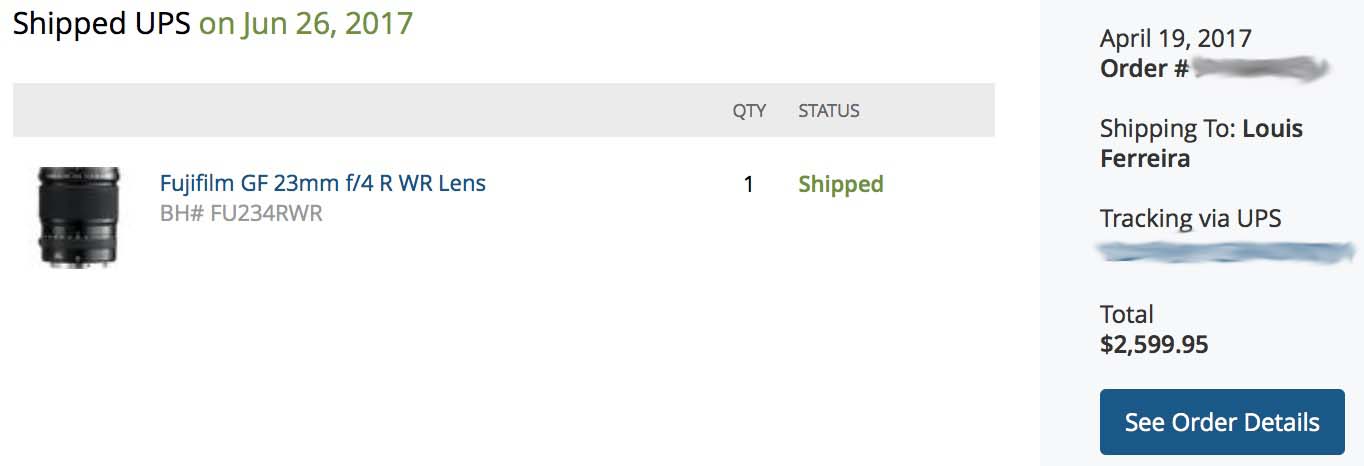Here is the reformulated descriptive caption for the image:

---

The screenshot displays a shipping status screen for a Fujifilm GF 23mm F-4RWR lens. In the upper left-hand corner, there's a notation indicating the item was shipped via UPS on June 26, 2017. A gray bar beneath this shows the headings "QTY" and "Status" in black text. Below the bar, the details of the shipped item are presented: An icon of the lens stands vertically accompanied by its description. The item has a serial number of BH# FU23-4RWR, displayed in gray text. It shows a quantity of 1, with the status marked as "Shipped". On the right side, the date April 19th, 2017 is noted alongside a partially blurred order number. The shipping is addressed to Lewis Ferraria, with the UPS tracking number also blurred out. The total cost of the item is $2,599.95. In the lower right-hand corner is a button labeled "See Order Details", in white text on a blue background. The entire information appears on a white screen presented in a narrow rectangular format.